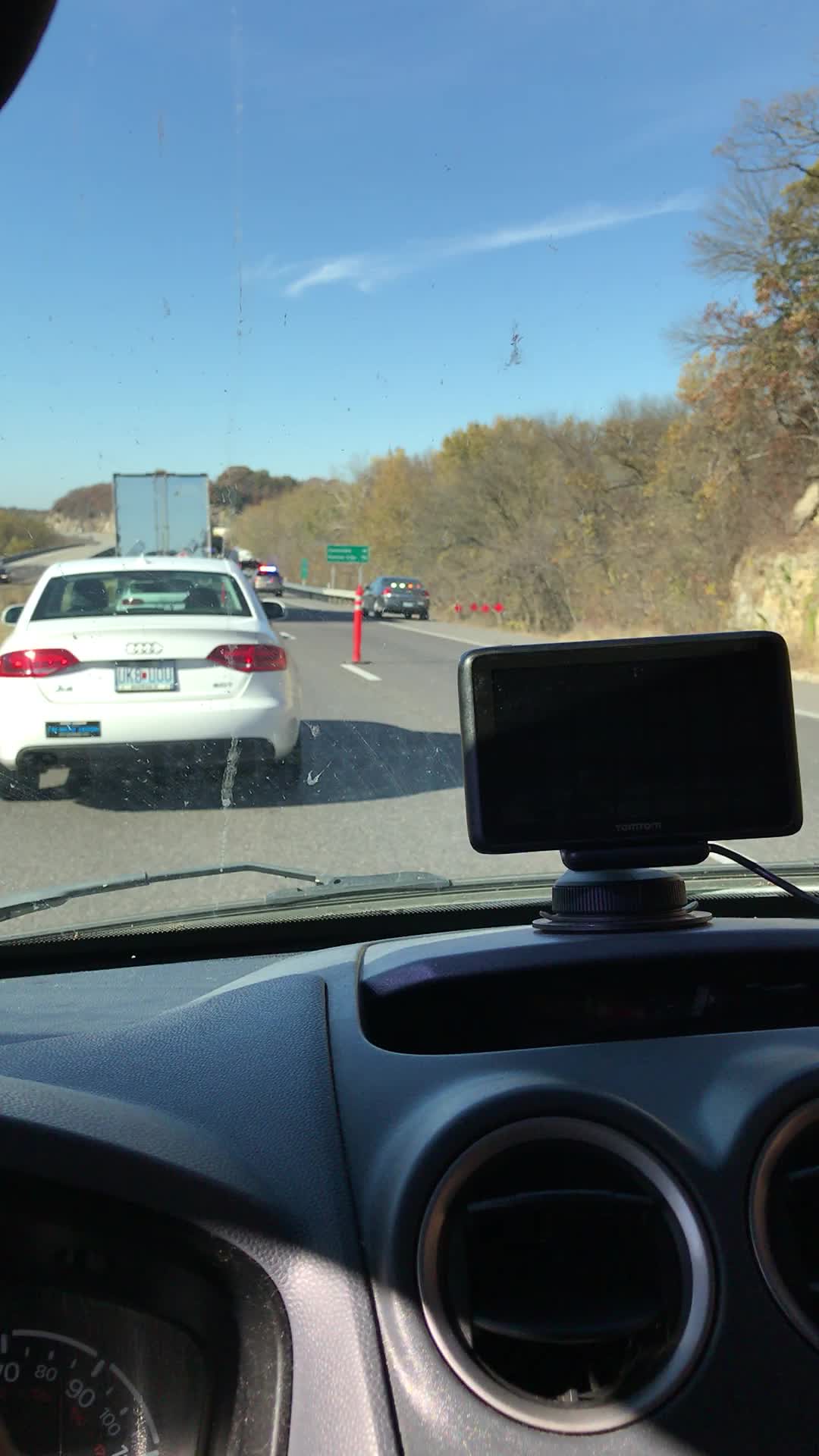The image captures a scene from inside a car during the daytime, viewed through the front windshield. The dashboard is partially visible, featuring air vents and a mounted smartphone, which is black with a charging cord attached. Off to the side, several red cones indicate ongoing construction work. In the distance, a green highway sign is visible, though its text is indiscernible due to the distance. Directly ahead, a white car is seen, suggesting traffic is slowing down. Additionally, a small portion of the windshield wiper is visible at the edge of the frame. Notably absent from the view are any people or the car's steering wheel.